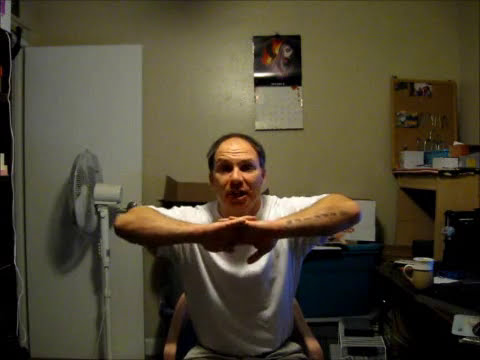In this slightly blurry and grainy color photograph, potentially a screenshot from an old video, a man with black hair is seated in an office chair, positioned centrally in his office. He wears a white T-shirt and has his fingers intertwined just below his chin, with his bent elbows pointing outward, seemingly in the middle of an exercise or stretch. His mouth is open as if mid-sentence. Behind him, on the light pea green wall, there is a calendar with a picture above it. The surrounding area appears cluttered, featuring a black desk with a computer monitor and coffee cup to the right, and a shelf nearby. To the left of the man is an open white door, and in front of it stands an oscillating floor fan.